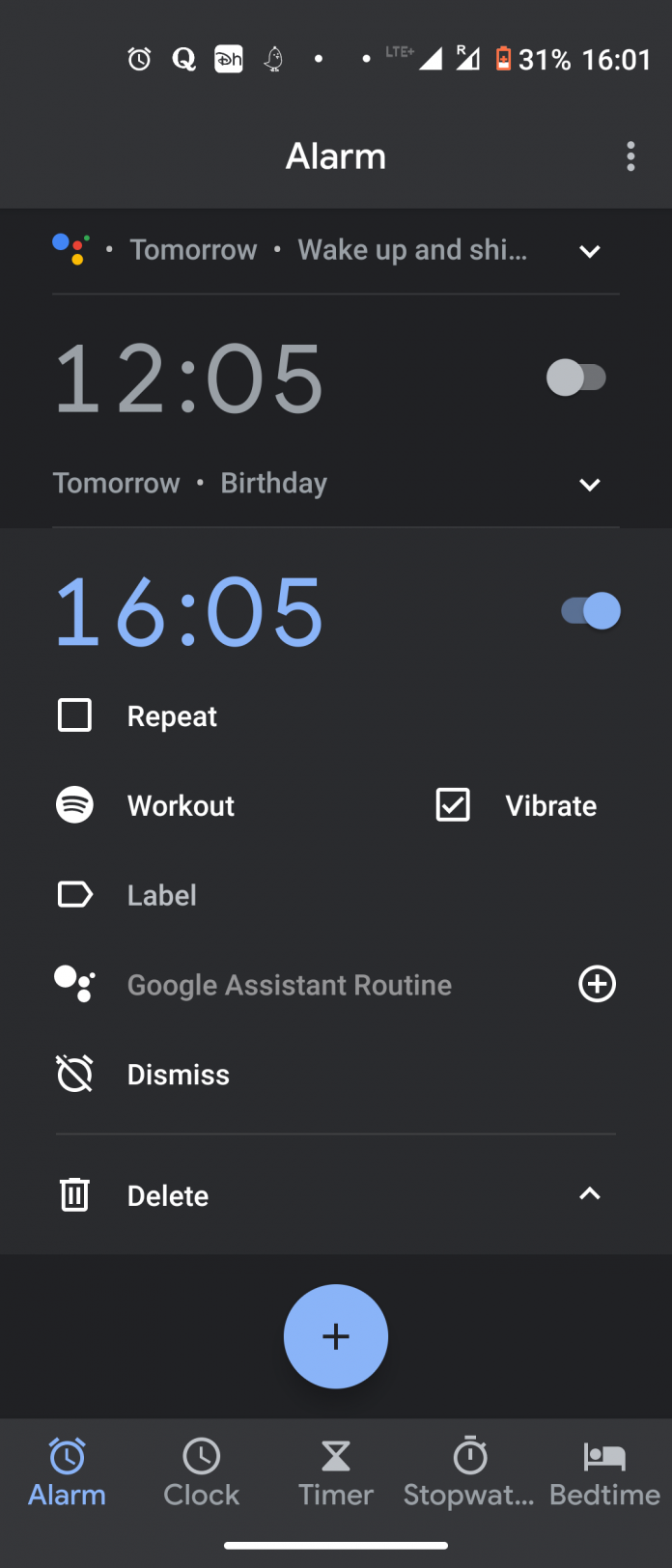This is a detailed description of an alarms page screenshot from a cell phone. The top inch and a half of the screen has a dark, almost black-gray background. Starting from the left, the top bar displays the current time, 16:01, in white text, followed by the battery level at 31%, with the battery icon shown in red. The network indicators follow: three out of four bars for mobile internet, a full Wi-Fi signal, and two white dots side-by-side. Next to these, there is a notifications icon and a small white square with "DH" written in black inside it. Further along is a white "Q" icon, followed by a white alarm clock icon.

Below this top bar, in the center in bold white text, it says "Alarm." On the right side, three gray buttons are vertically aligned. 

The main screen, about two inches in height, has a black background. At the top-left corner, there's a blue circle, followed by a red circle to its right, and a yellow circle below the red circle. Next to these, in gray text, it reads "Tomorrow," followed by a dot, then "wake up and sh…" and a greater-than sign pointing downwards.

In large gray text, "12:05" is shown, indicating an alarm time which is toggled off, with the toggle switch situated on the right side. Below this, it says "Tomorrow" followed by "Birthday" and another greater-than sign pointing down.

The subsequent part is detailed by a gray border enclosing a large blue alarm time, "16:05," which is toggled on from the right side. Adjacent to it is a black square with a white border labeled "Repeat." To the right, there are four icons and accompanying texts. One label reads "Work out," with a black square next to it featuring a white border and a white checkmark inside that says "Vibrate." The next entry is "Google Assistant Routine," followed by a white-bordered black circle featuring a white plus sign.

Toward the bottom, the options "Dismiss" and "Delete" are displayed. Additionally, there's another black-bordered section with a blue circle and a black plus inside it.

At the very bottom, a dark gray bar contains icons for different functions: "Alarm" (highlighted in blue), "Clock," "Timer," "Stopwatch," and "Bedtime" (all in white).